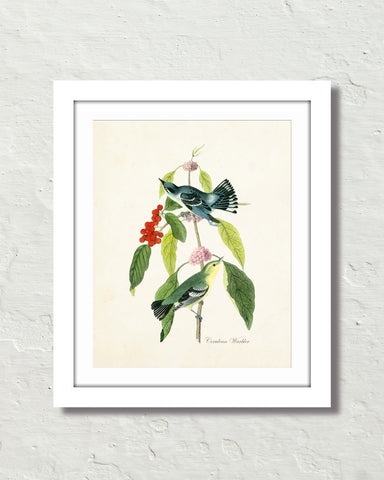The framed art piece, with its white frame and white mat, is set against a textured white wall. The background of the artwork is cream-colored. It features two intricately drawn birds perched on a branch adorned with foliage and berries. The branch sports small pink flowers in the middle and clusters of red berries on the left side, accompanied by a mix of dark and light green leaves. The bird on the top has a blue back with white and black stripes, a white belly and neck, and blue feet with a black beak. Meanwhile, the bird on the bottom is characterized by its green back with white and black stripes, a light green head, and blue feet with a black beak. At the bottom of the piece, there's a signature, though it is indecipherable.